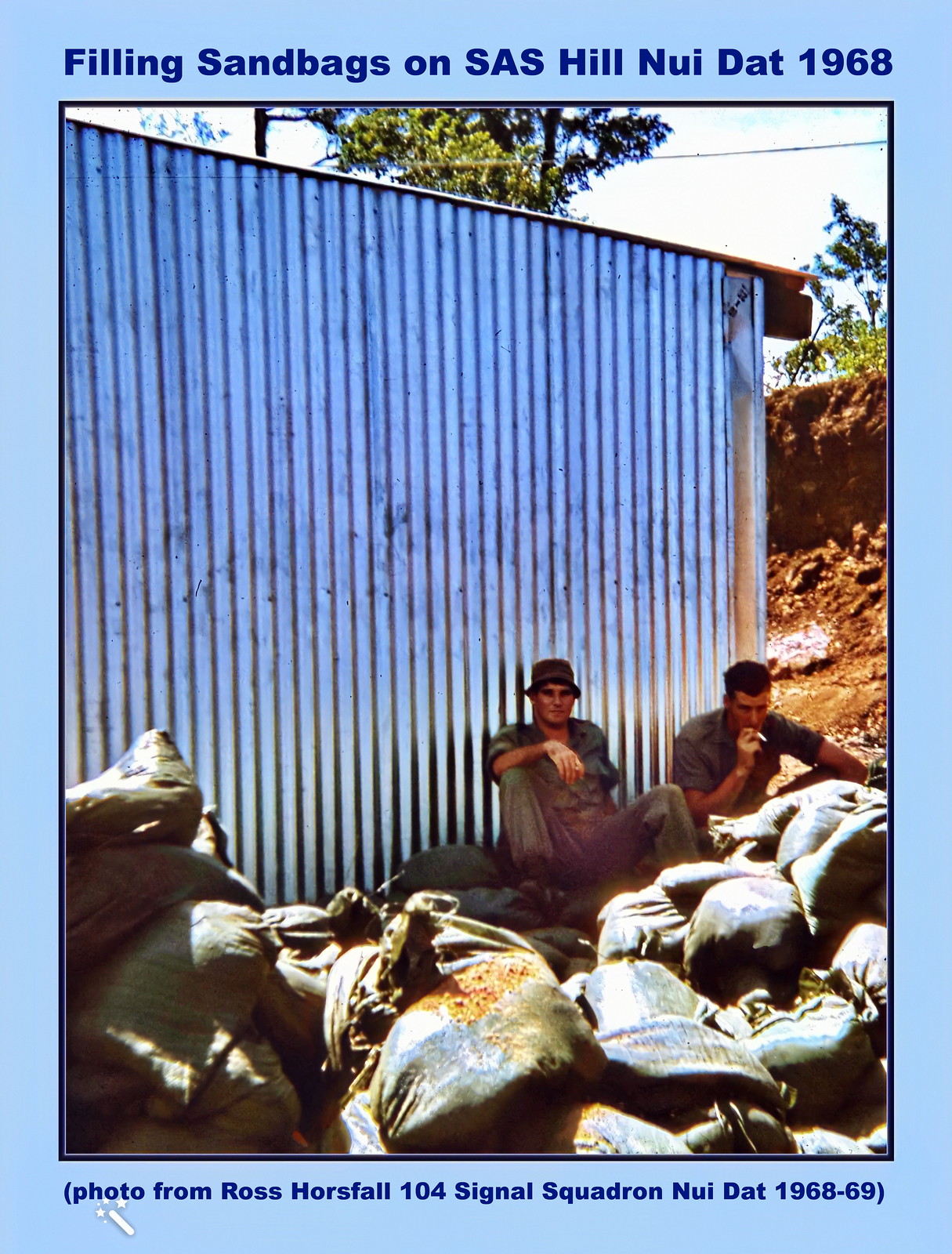This slightly faded photograph, set in Vietnam, is framed by a light blue border with bold, dark blue text. At the top, it reads, "Filling Sandbags on SAS Hill, Nui Dat, 1968." The bottom text states, "Photo from Ross Horsefall, 104 Signal Squadron, Nui Dat 1968-69." Inside the thinner inner blue border, the central scene captures two men, dressed in green military uniforms, sitting beside an untidy pile of large sandbags in shades of gray and brown. The man on the left, wearing a hat, leans against a corrugated metal wall, while the man on the right smokes a cigarette. Behind them is a dirt field with scattered trees and power lines. The sky above is slightly overexposed, suggesting the image was taken outdoors in the middle of the day.